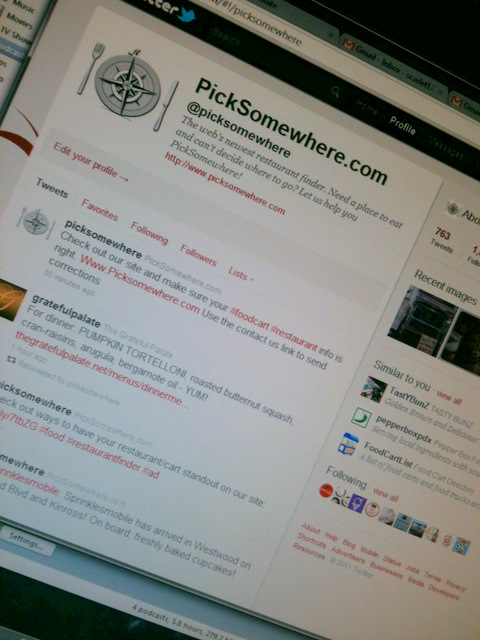This image features a slightly tilted computer screen displaying the website "picksomewhere.com," which is branded as the web's newest restaurant finder. At the top, "PickSomewhere.com" is prominently displayed, along with the tagline: "Need a place to eat and can't decide where to go? Let us help you pick somewhere." Alongside this text, there is an image of a plate serving as a compass, flanked by a fork and knife. Below, the screen shows various user account details such as tweets, favorites, following, followers, and lists. A link to the Grateful Palate restaurant is highlighted, detailing a dish of pumpkin tortilla, roasted butternut squash, cranberries, arugula, and bergamot oil. Additional links and advertisements are visible but hard to decipher on the right side of the screen. The photo of the screen appears to be taken at an angle, perhaps with a phone or camera, giving an off-centered, askew appearance.